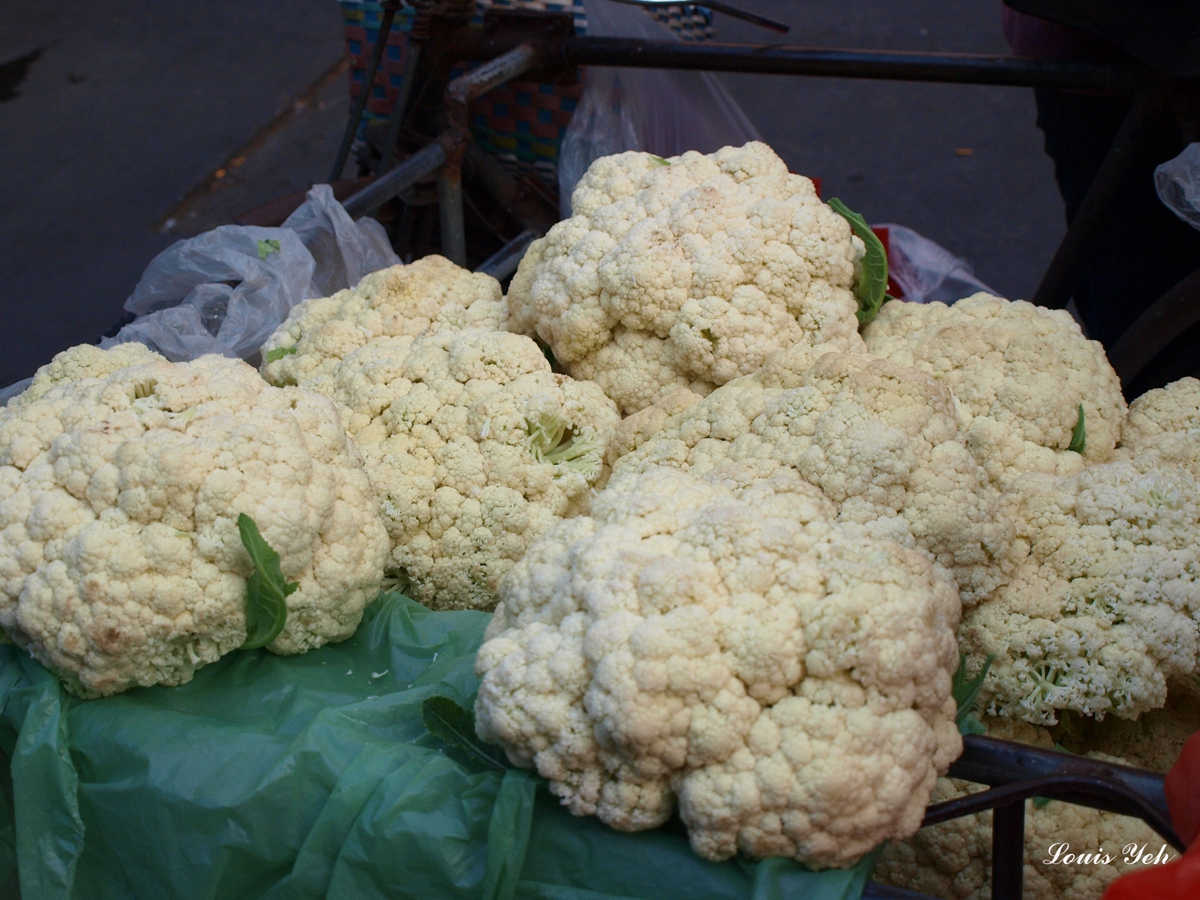The image depicts a collection of large heads of cauliflower, approximately eight or nine in total, placed on what appears to be an industrial rack or cart. The cauliflowers, predominantly white with a few green leaves remaining, seem freshly harvested and are prepared for processing or packaging. They rest on a tray that is covered with a green plastic fabric or bag, complemented by additional white and red plastic bags in the vicinity. Metal bars along the sides and back suggest the cauliflowers are contained within a cart. Noteworthy details include a small bit of text in cursive white lettering, "Lewis Y-E-H," located in the bottom right corner. The background also features some indistinct items, with traces of orange and blue visible. Overall, the cauliflowers are densely packed together, displaying a slightly oxidized appearance in spots but largely appearing full and robust.